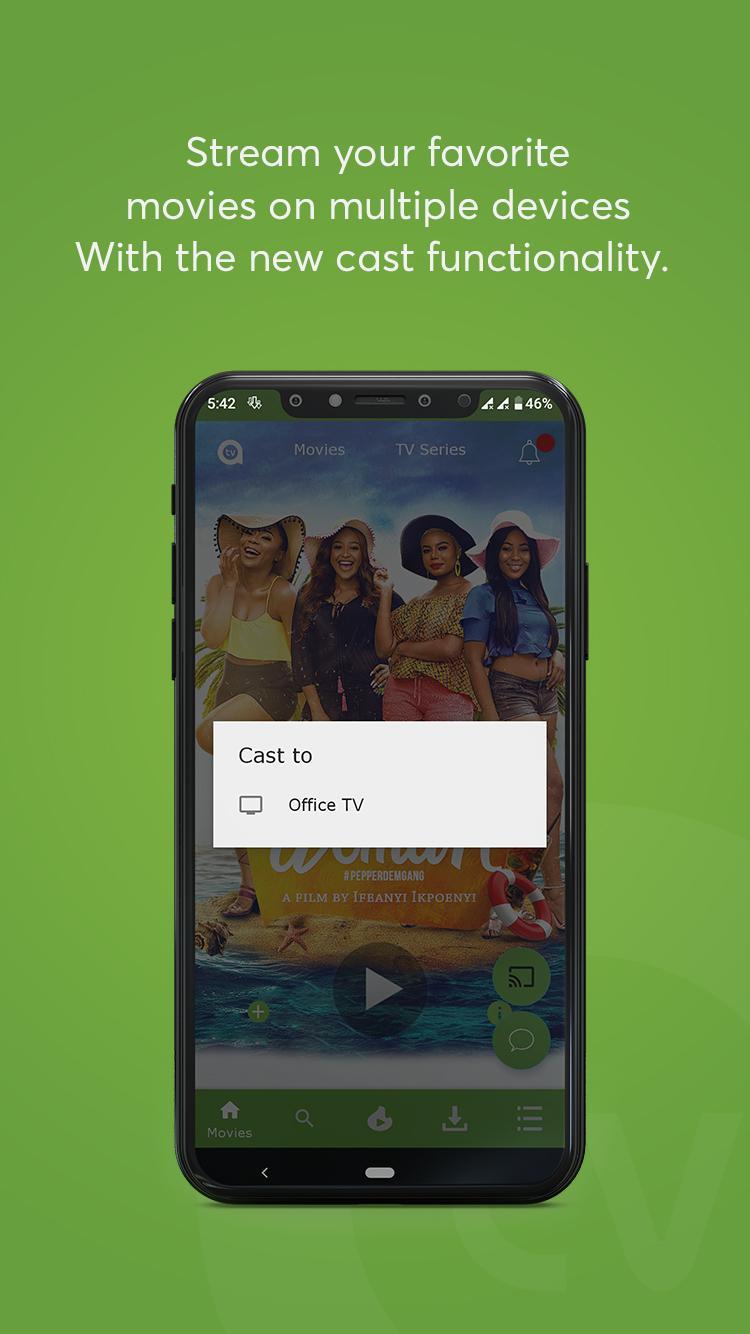**Caption:** 

In this vibrant advertisement, a cutting-edge iPhone is showcased prominently, highlighting its new casting functionality. The background features a dynamic blend of dark green and lime green hues, creating a visually striking canvas for the central message. The ad’s text is in crisp white font for high contrast and readability. The iPhone displays a pop-up window that says "Cast 2," indicating a connection to "Office TV." On the iPhone screen, there's a scene from a TV show featuring four women, all donning stylish hats, though the show's title is obscured by the pop-up. The headline boldly promotes: "Stream your favorite movies on multiple devices with the new cast functionality." This advertisement, perfectly suited for viewing on phones or at the mall, emphasizes the convenience and versatility of streaming media across various screens.